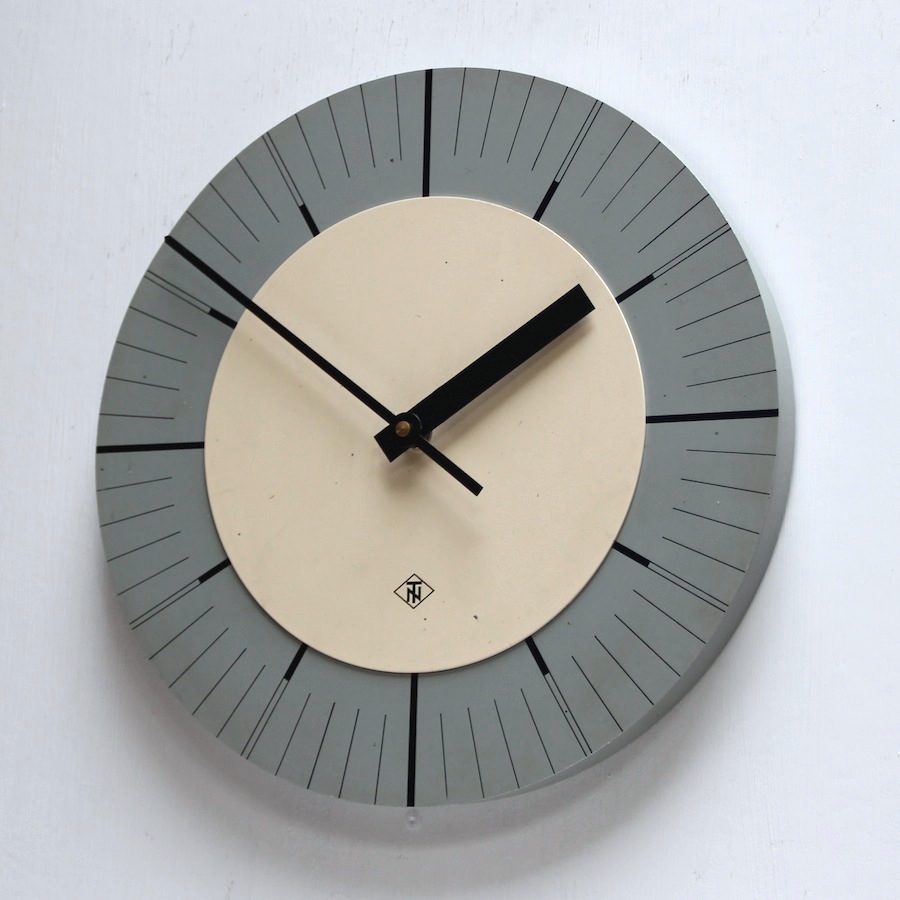The image features a simple, modern wall clock mounted against a plain white wall. The clock casts a subtle gray shadow below it. Its design is minimalistic and sleek, with no numbers on the face. Instead, the outer ring is a pale medium gray adorned with black hash marks. Four of these hash marks—indicating the 12, 3, 6, and 9 positions—are darker, thicker, and extend slightly longer. 

The inner circle of the clock is a cream or tannish off-white color, adding a subtle contrast to the outer ring. The black hour and minute hands are distinct, with the hour hand being shorter and thicker and the minute hand longer and thinner, currently showing a time of 1:51. A small, unobtrusive logo featuring a diamond shape with a superimposed T and N appears near the bottom of the inner circle.